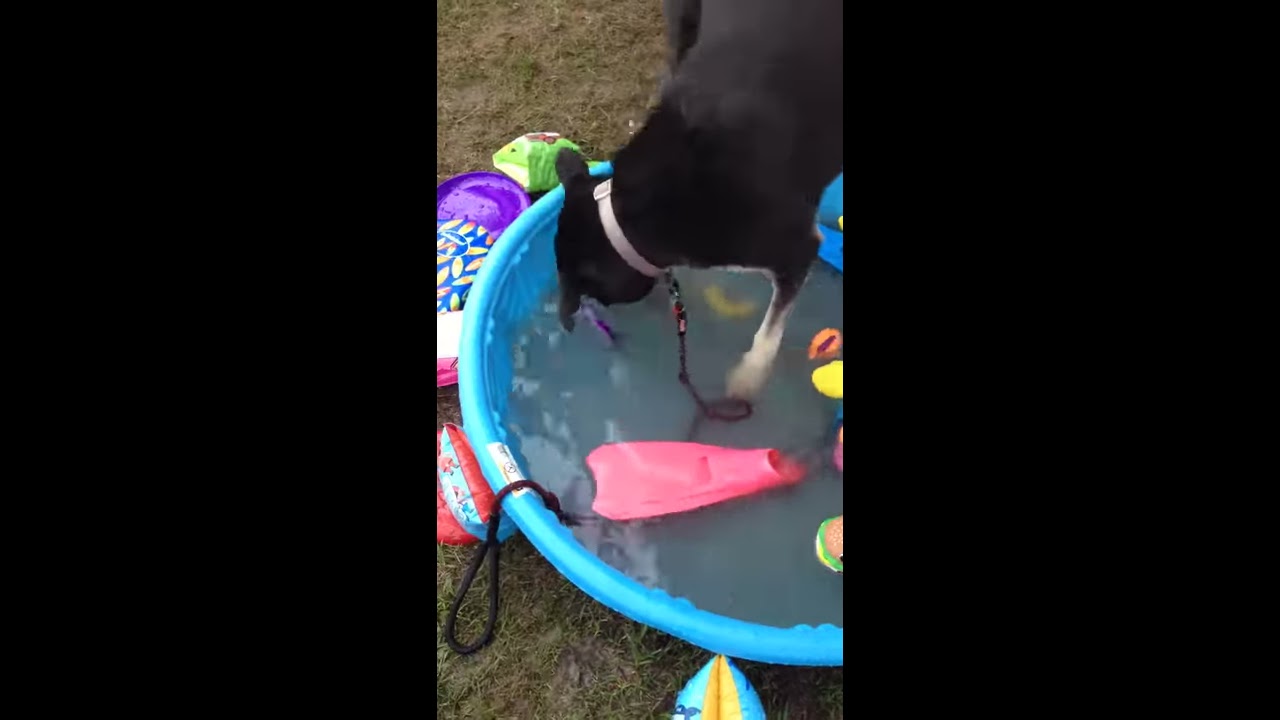In this outdoor daytime photograph, a black dog with white legs is standing in a light blue plastic kiddie pool filled with water. The dog, which has a collar and a dangling leash partially submerged in the water, appears to be drinking or searching for something in the pool. Scattered around and inside the pool are numerous colorful toys, including a pink flipper, yellow, orange, green, red, blue, and purple objects. The ground surrounding the pool is a mix of green grass and brown earth. The image features vertical black strips on both the left and right sides, and only the front half of the dog's body is visible in the frame.